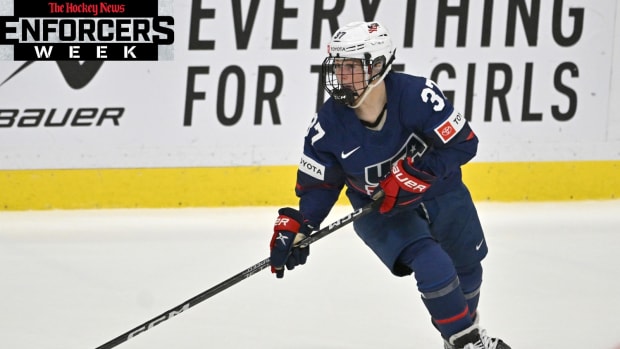This image captures a hockey player standing on the ice during what appears to be a women's ice hockey tournament. The player is outfitted in a navy blue jersey adorned with the number 37 and sponsor logos, including a prominent white Nike logo. They are well-equipped with blue shorts, blue shin guards, and red and blue Bauer gloves. Their distinctive white helmet features a black wire face mask for protection. In their hands, they grip a black hockey stick. The backdrop of the image reveals a white advertisement barrier with a yellow vertical bar, and black lettering that reads "Everything for girls." In the upper left corner, a black box with red text reads "The Hockey News," while below it, white and black text states "Enforcers Week." The scene is set on a pristine white ice surface, evoking the intensity and ambience of the hockey arena.